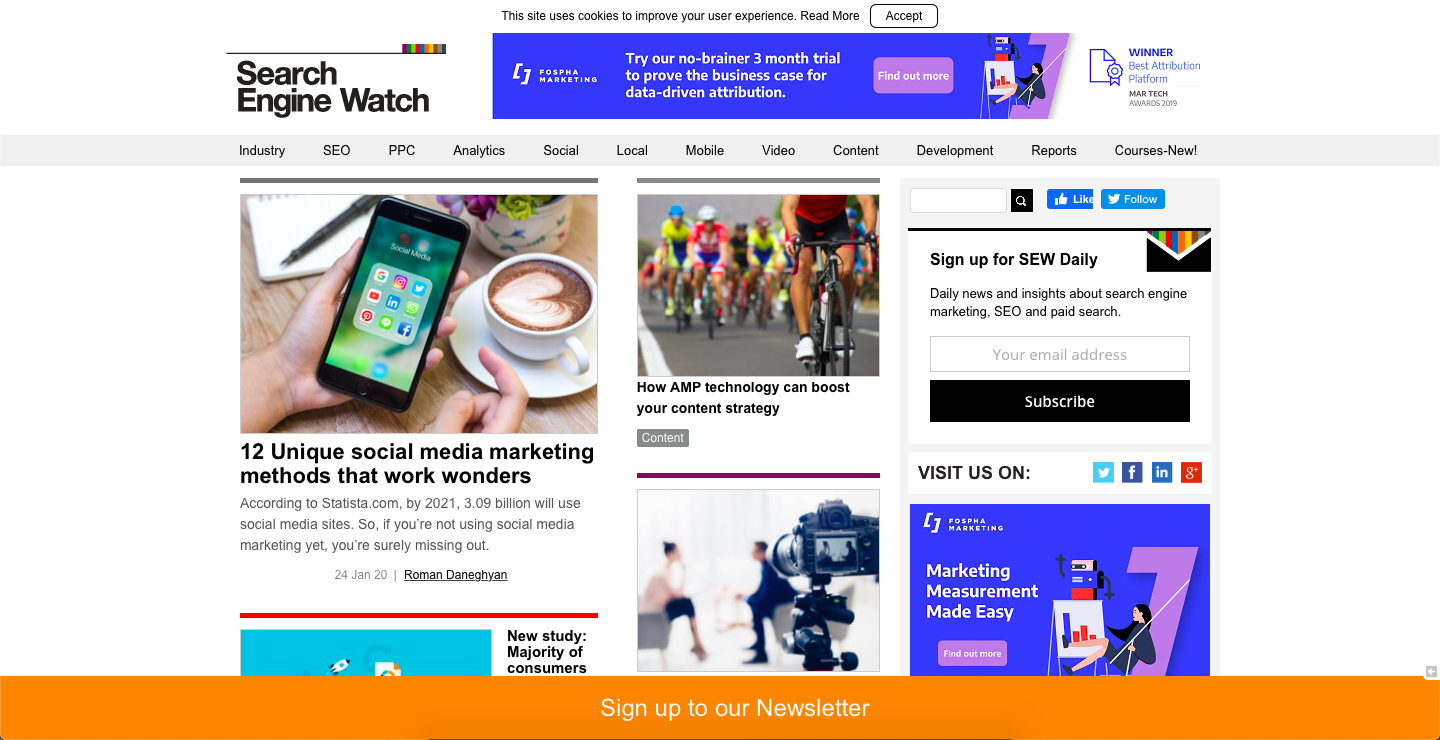This image features a promotional advertisement for a search engine marketing service, highlighted by a prominent headline reading, "Try our no-brainer three months trial to prove the business case for data-driven attribution." Below this, there's a call-to-action button prompting viewers to "Find out more."

Adjacent to the main advertisement are additional sections resembling blog posts or sponsored articles. The first article on the left is titled "12 Unique Social Media Marketing Methods," which indicates that, according to Statista.com, by 2021, an estimated 3.9 billion people will use social media. The article emphasizes that not utilizing social media in marketing strategies is a missed opportunity.

Another highlighted item is an article discussing a "New Study of Majority Consumers" and a piece on "How MP Technology Can Boost Your Content Strategy." The image also includes a sign-up prompt for "SU Daily," a newsletter offering daily news and insights about search engine marketing, SEO, and paid search.

The overall layout is designed to not only promote the trial offer for data-driven attribution but also to engage viewers with additional content on social media marketing strategies and industry insights.